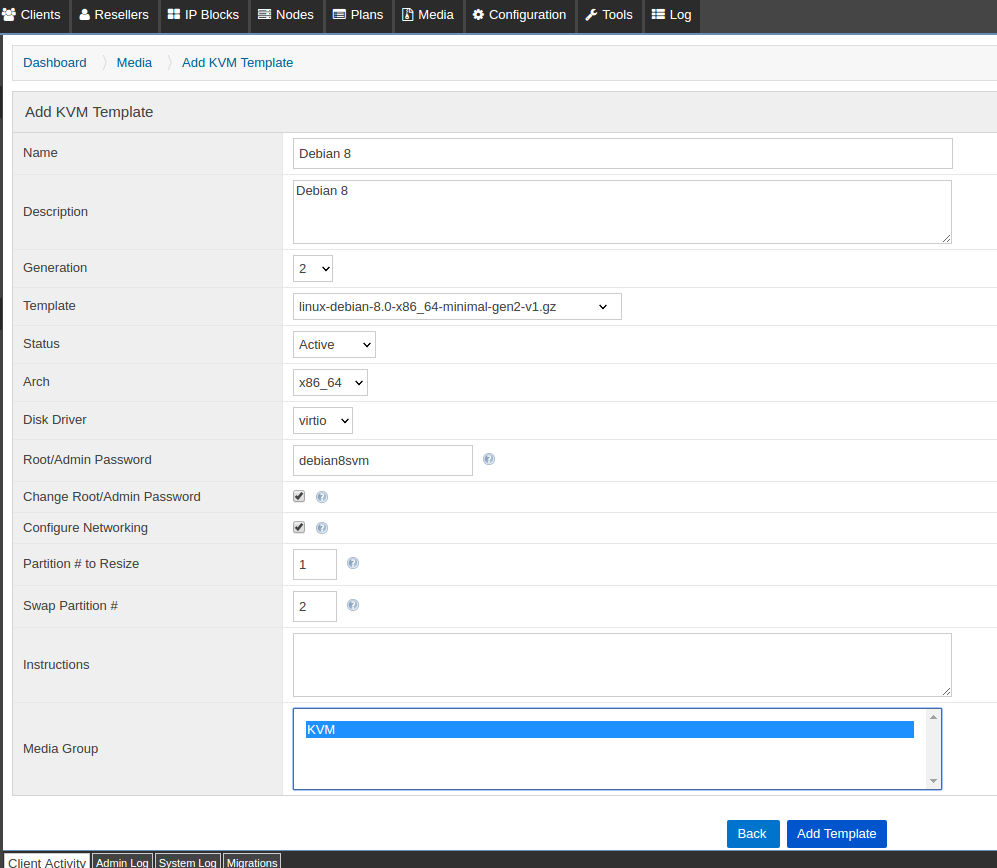A screenshot capture depicts the interface of a website, emphasizing its intricate layout and detailed menus. At the very top is a diminutive logo, too small to discern the site's identity. Directly below the logo is a sleek, black menu bar featuring white-font hyperlinks to sections such as "Clients," "Resellers," "IP Blocks," and "Nodes," providing quick navigation to these areas. Underneath this main menu, there is a secondary navigation bar highlighting options like "Dashboard" and "Media."

The focal point of the image is the "Add KVM Template" section, which has been activated by the user. This section expands to reveal an extensive form designed for entering various pieces of system information. The form includes fields for the system's name (non-personal, technical identifiers), a detailed description, and the generation of the system. It's evident that completing this form requires entering a substantial amount of technical data, suggesting that the website is geared towards users involved in programming or IT infrastructure management. The detailed nature of the form indicates a high level of specialization and technical expertise necessary for its completion.